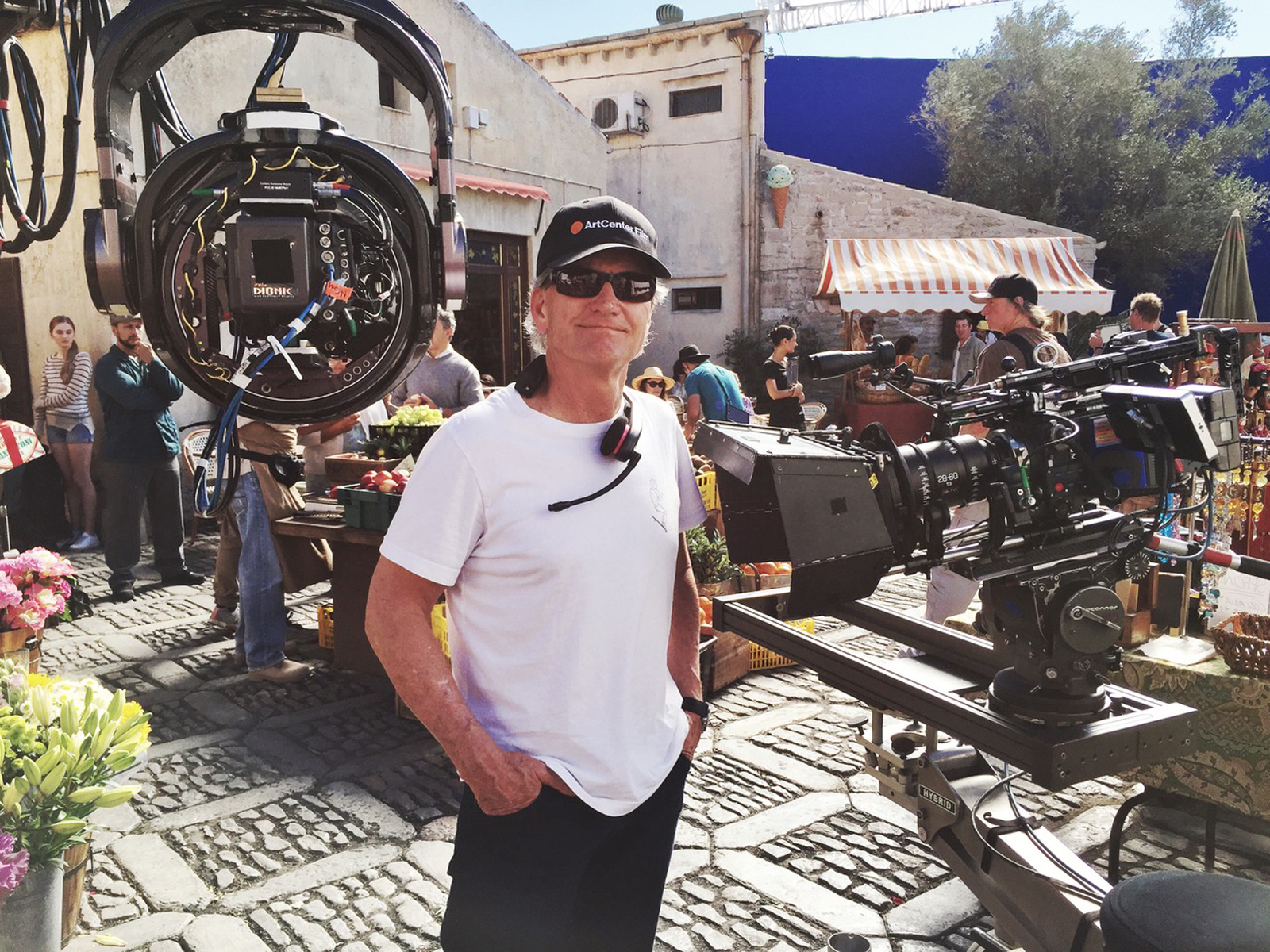This horizontally-aligned, outdoor photograph captures what appears to be a small event on a movie set. The ground consists of gray rectangular pavers with small chunks of rock embedded in them. At the forefront stands a man in a white short-sleeved t-shirt, black shorts or pants, and a black baseball cap with "Art Center" partially visible. He has a headset with a microphone around his neck, wears black sunglasses, and sports a black watch on his left wrist. His hands are in his pockets, and he smiles at the camera with his mouth closed, revealing some white hair escaping beneath his cap.

Behind him, various individuals, mostly men, are engaged in different activities. To the man's right, there is a large, expensive-looking movie camera mounted on a swinging arm, with an attached seat for operation. This setting, which seems to depict an older-looking building that might resemble a café in a rugged environment, adds character to the scene. In the upper left, a woman wearing jean shorts and a striped long-sleeved shirt stands beside a tan stone building with a striped orange and white canopy. Several tables with fruit, possibly apples, hint at either a place for people to grab a snack or part of the movie set. The sky is clear blue without any clouds, visible just at the top of the image.